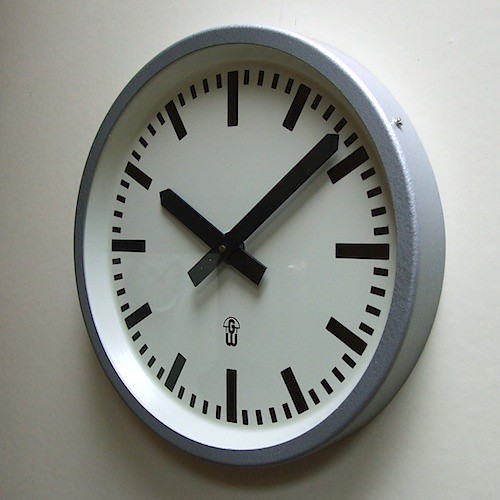This is a detailed, edited caption: 

A color photograph of a minimalist wall clock mounted on a pristine white background. The round clock features a sleek gray metal rim enclosing its face. Instead of traditional numbers, the hours are marked by long, thin rectangles, with each minute denoted by very short dark rectangles. The clock's time is captured at 10:08, as indicated by its distinctive black arrow-shaped hour, minute, and second hands. Nestled beneath the central clock hands is a logo displaying the initials "G" and "W," artfully aligned atop one another.